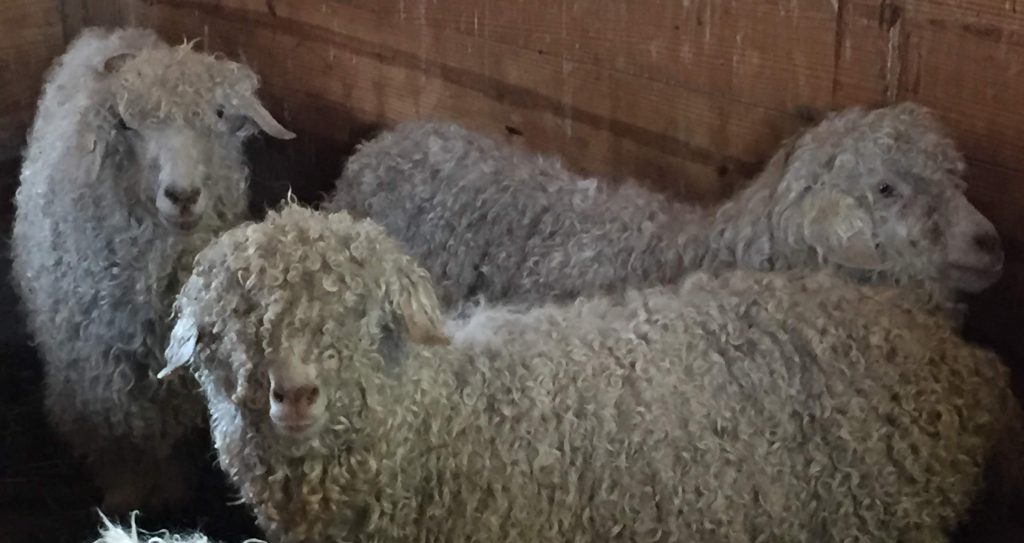The image shows a close-up of three raggedy, grey sheep standing in a pen inside an old barn. Their coats are long and curly, with one sheep in the center having its eyes almost completely covered by its fur. The sheep to the left and center are looking directly at the camera with closed mouths, while the third sheep on the right is gazing off to the side. The barn appears aged, with wooden walls that have a reddish to pinkish hue. Additional fur is visible in the foreground, suggesting the presence of another sheep just out of the frame. Despite the low quality of the image, the distinct features of the sheep, including their black-tipped white noses, can be seen.